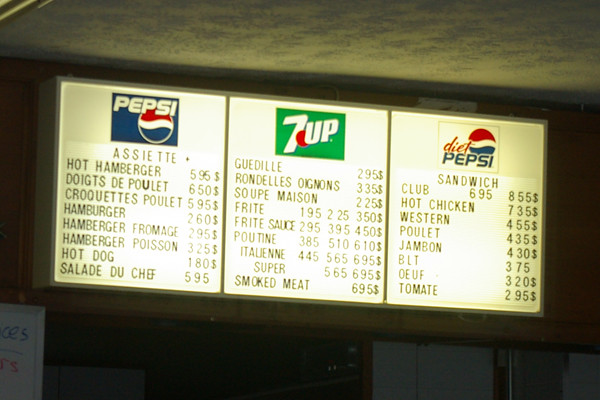This illuminated rectangular signboard, likely positioned indoors, serves as a detailed menu display. The signboard is divided into three distinct sections, each highlighting different items and logos.

The left section features the iconic Pepsi logo at the top, followed by the word "Assiette" in bold black letters. Beneath this heading, an array of menu items are listed, predominantly in French. These include "Hot Hamburger" (notably misspelled as "Hamberger"), "Doigt de Poulet" (Chicken Fingers), "Croquettes Poulet" (Chicken Nuggets), correctly spelled "Hamburger," incorrectly spelled "Hamberger," "Fromage" (Cheese), "Hamburger Poisson" (Fish Burger), "Hot Dog," and "Salade du Chou" (Coleslaw).

The middle section showcases the 7UP logo, characterized by its green, white, and red colors. This section continues the trend of presenting menu items primarily in French, with the exception of "Smoked Meat" at the bottom. Notable among the listed items is "Poutine," suggesting that this menu belongs to an establishment located in a French-speaking region of Canada.

The right section displays the Diet Pepsi logo in its recognizable red, white, and blue color scheme. Below this, the heading "Sandwich" introduces various sandwich options available to customers.

The entire signboard is edged with a gray and brown border, enhancing its visibility against the backdrop. The white ceiling above the signboard reflects natural sunlight, further illuminating the menu's contents for easy reading.